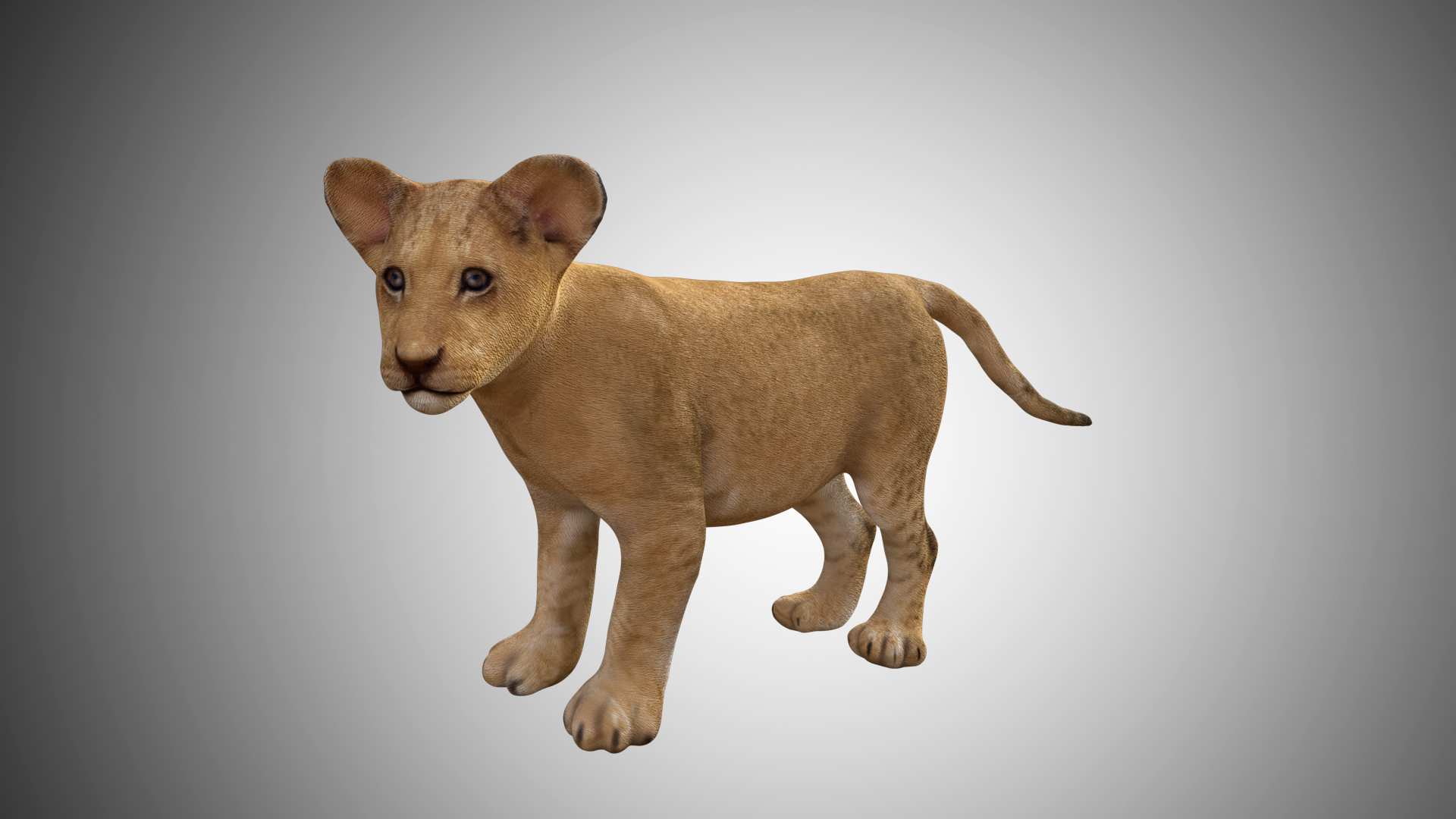This is a detailed digital image, possibly a CGI rendering, of a muscular lion cub standing on four legs. The background features a subtle gradation from white to gray, becoming darker towards the edges, giving a portrait-like appearance rather than a natural setting like a jungle. The cub has a coat of light brown fur, with its legs adorned with white fur splashed with faint brown spots. Its medium-sized tail, covered in short fur, is light brown at the base and gets darker towards the tip. The lion cub's ears are large, short, and rounded with a pinkish hue inside. It has a white chin and a somewhat expressionless face with dark, contemplative eyes. The overall posture of the cub is slightly turned to the left, with its head angled further left, giving it a poised yet inquisitive look.